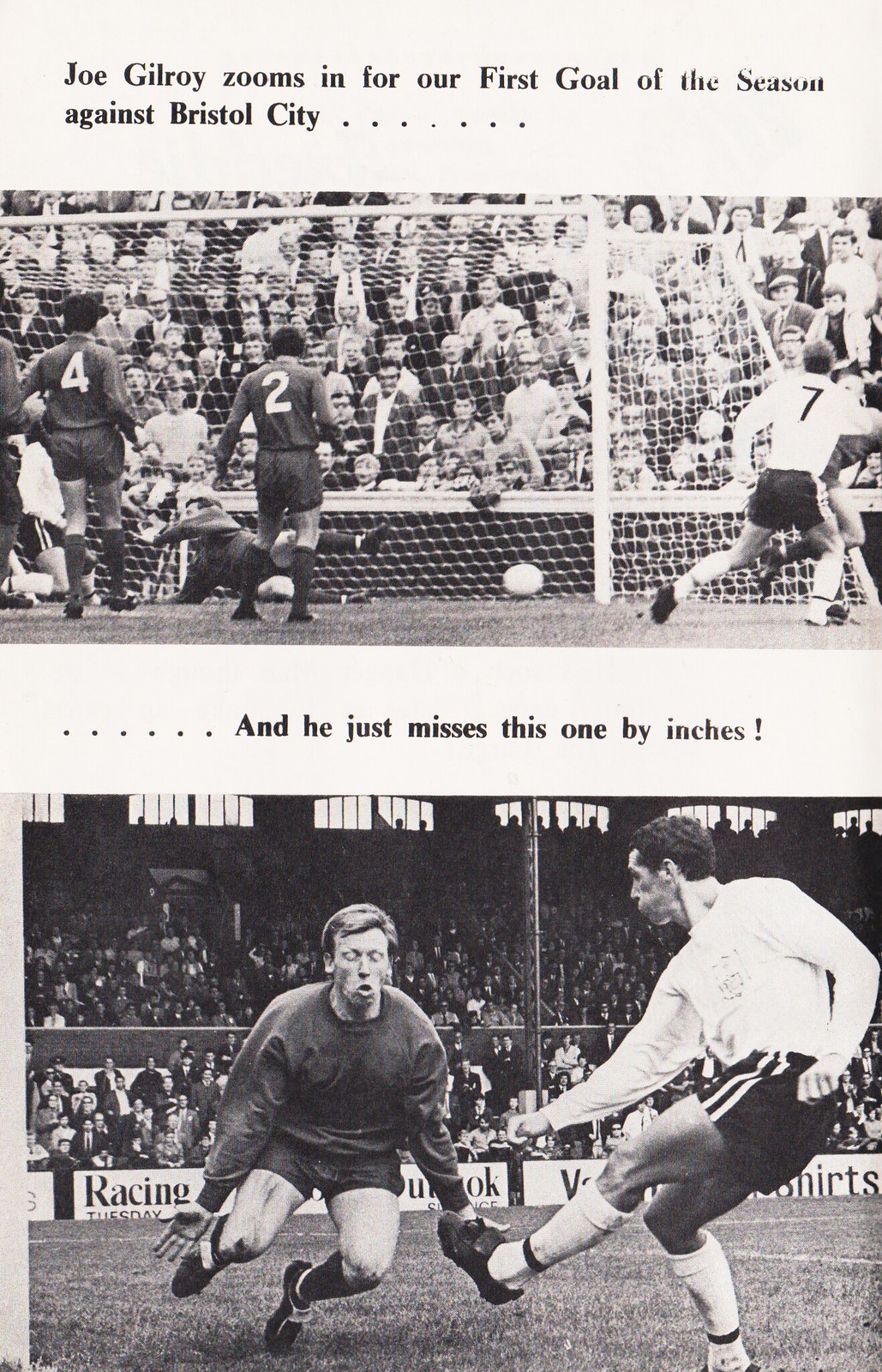The image depicts a newspaper or magazine article set against a white background with black text. The page features two black and white photos of a soccer game, one above the other. The top section of text reads, "Joe Gilroy zooms in for our first goal of the season against Bristol City." Below this text is a photograph showing a dynamic moment where a soccer ball has just been kicked into the goal. In this image, players can be seen running on the soccer field, with one player falling to the ground and a large crowd of spectators filling the stands. Two players in this scene are wearing dark uniforms, one with the number four and another with number two, while a number seven player is positioned to the right of the net.

The second photo has accompanying text that says, "And he just misses this one by inches." This image captures two soccer players in action: one player in a dark uniform appears to be diving toward the ball, while another player in a long white-sleeve shirt and dark shorts looks set to kick it. The background of both photos includes visible barricades adorned with company logos and a crowd of onlookers, further emphasizing the high-energy atmosphere of the soccer match.